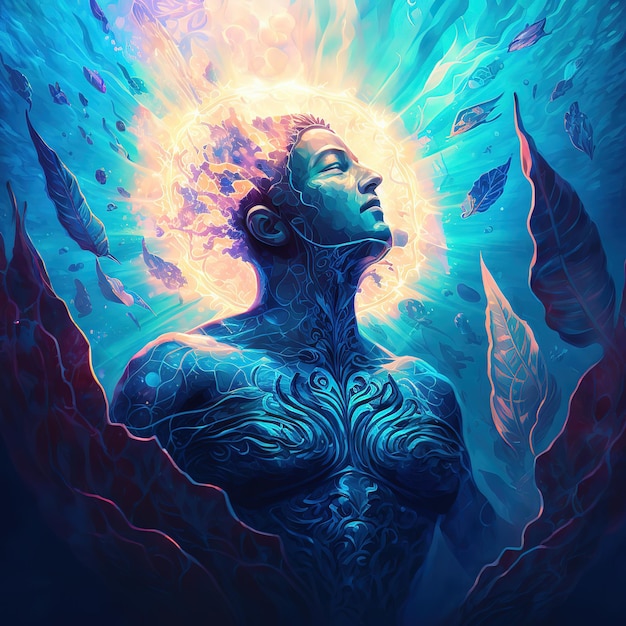The digitally-created image features a humanoid figure, centrally positioned and depicted from the stomach up. The figure, predominantly male in appearance, has a body and skin comprised of a swirling blue, almost otherworldly material interspersed with carved patterns and curl designs, suggesting a blend between a human and an android or perhaps a mystical being like a merman. His chest and shoulders are adorned with delicate carvings and thin lines that extend over his neck and to his chin. His eyes are closed, and his face is uplifted in a serene, almost transcendent pose, captured from a side profile. The back of his head scatters into small, colorful pieces that seem to merge and float into the surrounding image, creating an ethereal effect. A light yellow and very light pink aura of light emanates around his head. The background is filled with dark blue, with elements resembling water and seaweed-like leaves floating around him, creating a cosmic, underwater atmosphere. The overall color palette employs various shades of blue with touches of yellow, pink, and purple, enhancing the mystical and nature-infused setting.